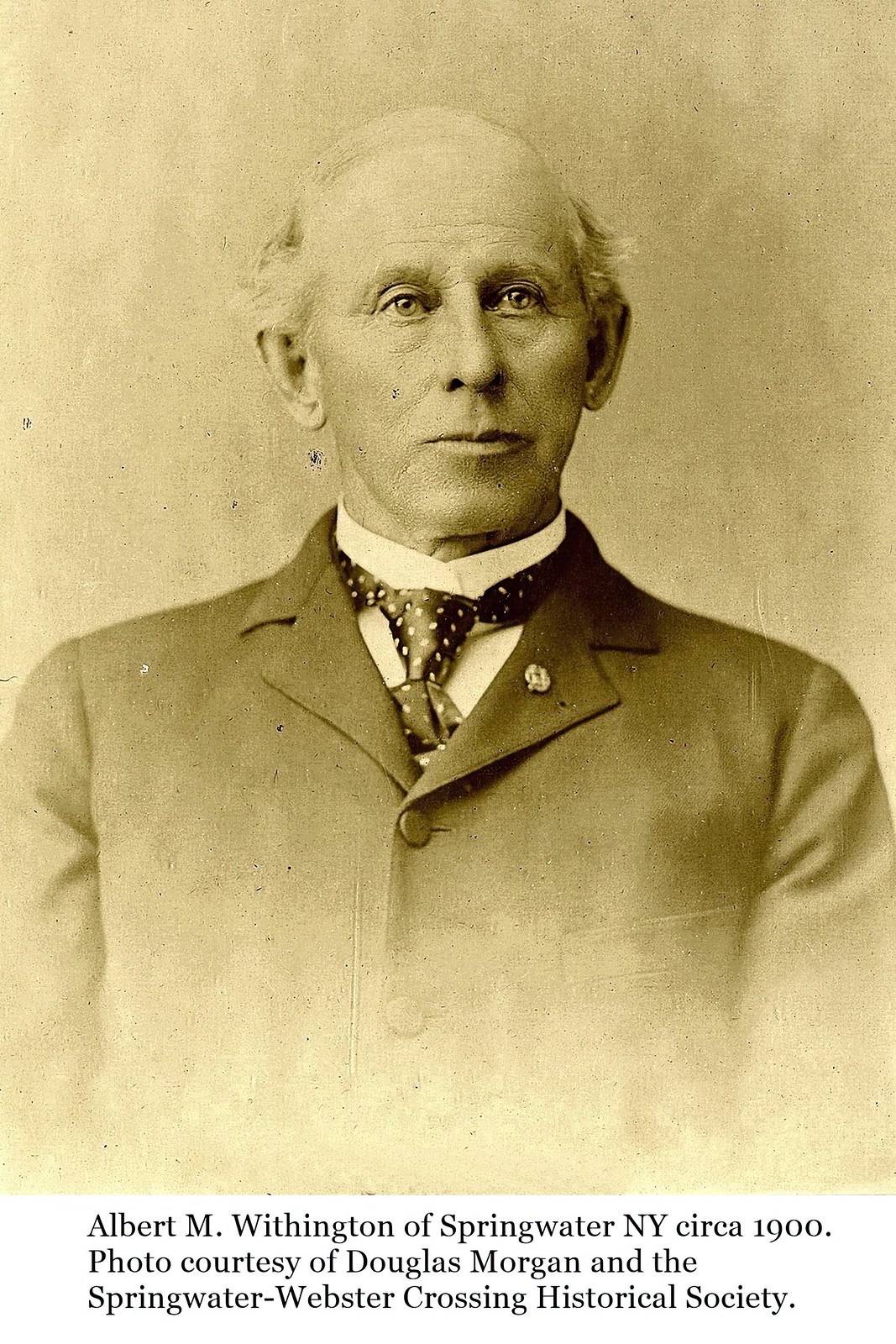This is a scanned image of a yellowed and worn black-and-white portrait from around 1900. The photograph depicts Albert M. Withington of Springwater, New York. Courtesy of Douglas Morgan and the Springwater Webster Crossing Historical Society, the text at the bottom reads, "Albert M. Withington of Springwater, New York, circa 1900."

In the portrait, Albert M. Withington, a man who appears to be in his late 50s or early 60s, is dressed in formal attire. He wears a dark jacket buttoned up to the tie, which is black with white polka dots, along with a white collared shirt. The man is partially bald with white hair on the sides of his head above his ears. He has blue eyes and pursed lips, and his head is turned slightly to the right. The photo has an orange hue due to its age and the degradation of the film. The backdrop appears to be a white or gray color, and the photograph has begun to fade at the bottom edges.